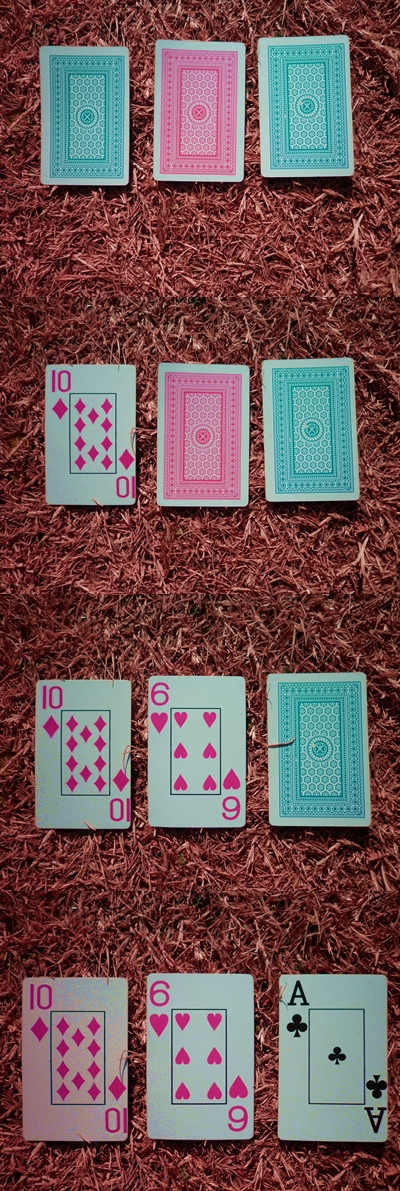The image depicts a sequence of cards laid out in four rows on a brown wood mulch surface, illustrating the progression of turning over the leftmost card in each subsequent row. 

In the top row, there are three face-down cards: the leftmost is blue, the middle is red, and the rightmost is blue. 

The second row features three cards: a face-up 10 of Diamonds on the left, a red face-down card in the middle, and a green face-down card on the right. 

The third row displays three cards: a face-up 10 of Diamonds on the left, a face-up 6 of Hearts in the middle, and a green face-down card on the right. 

In the bottom row, there are three face-up cards: a 10 of Diamonds on the left, a 6 of Hearts in the middle, and an Ace of Clubs on the right. 

This visual sequence suggests the step-by-step revelation of the cards, starting from the top row's leftmost card and proceeding down to the bottom row.